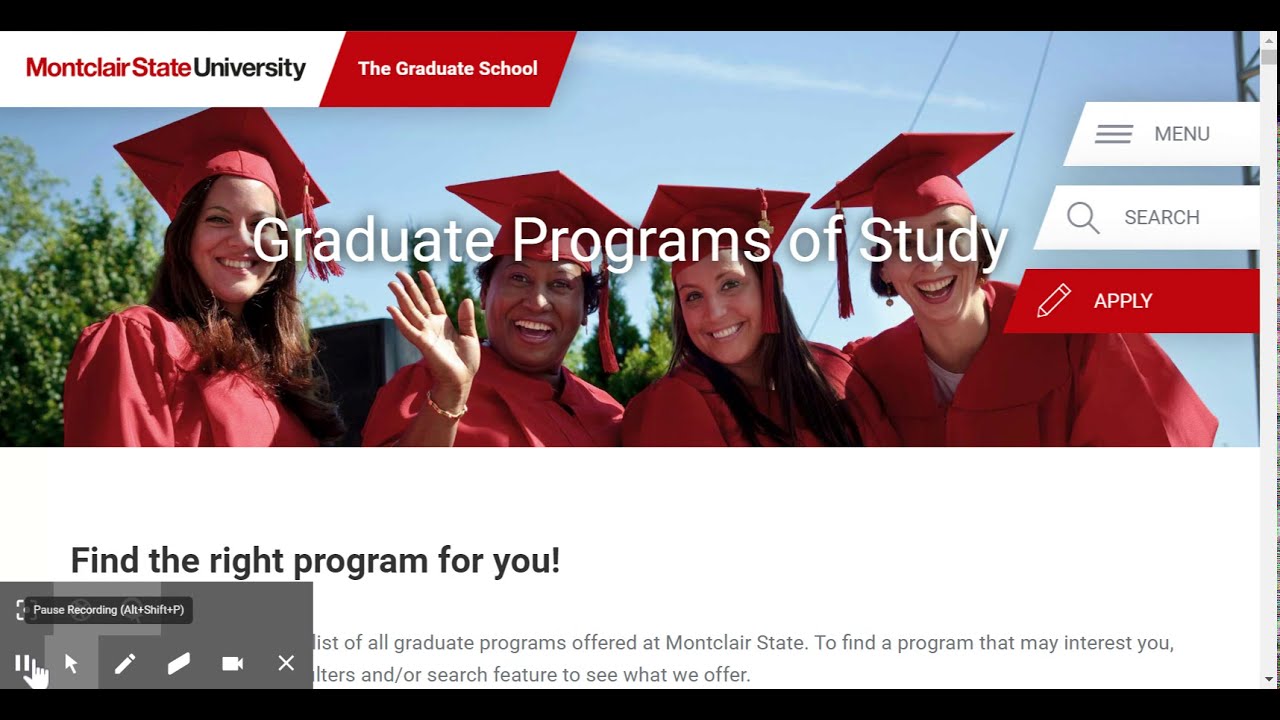This rectangular advertisement for Montclair State University features a prominent black border along the top and bottom edges. Positioned on the upper left of the main image, a notification reads "Montclair State University," accompanied by a red box with white text stating "The Graduate School." Four female graduates dressed in red caps and gowns are prominently displayed in the center, with one Black woman and three White women all smiling at the camera. Across the middle of the image, bold white text declares "Graduate Programs of Study."

On the far right, three interactive buttons are visible: a white "Menu" button, a white "Search" button, and a red "Apply" button with white text. Toward the bottom center, the phrase "Find the right program for you" is written to guide the viewer. In the bottom left corner, a small gray pop-up box displays various icons including a pause button, an arrow, a pencil, an eraser, a video camera, and an X, offering additional interactive options.